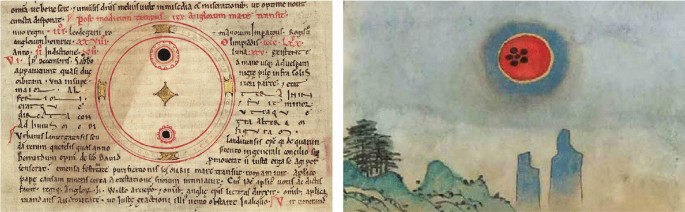This image consists of two distinct pictures side by side. On the left is a page from a book featuring text in a non-English language, incorporating both black and red ink, with a central circular symbol surrounded by writing. The main circle is red and open, marked at its north, south, east, and west points with yellow marks. Inside this open circle, there are two smaller circles, one larger with a black center situated at the top, and one smaller with a black center at the bottom. Additionally, a four-point star is placed within these circles.

To the right, there is a watercolor-style graphic that appears to depict a scene reminiscent of a Japanese sketch. The sky is a light blue with a darker blue circle at its center, within which sits a bright red circle containing a flower-like emblem, resembling a red bowling ball with black spots. This emblem floats above a gradient landscape that transitions to brown at the bottom. Silhouettes of two people in blue stand at the lower center of the image. To the left of these figures, a tree stands against a backdrop of mountains, likely rendered in watercolor, completing the composition with an evocative blend of blues and browns.